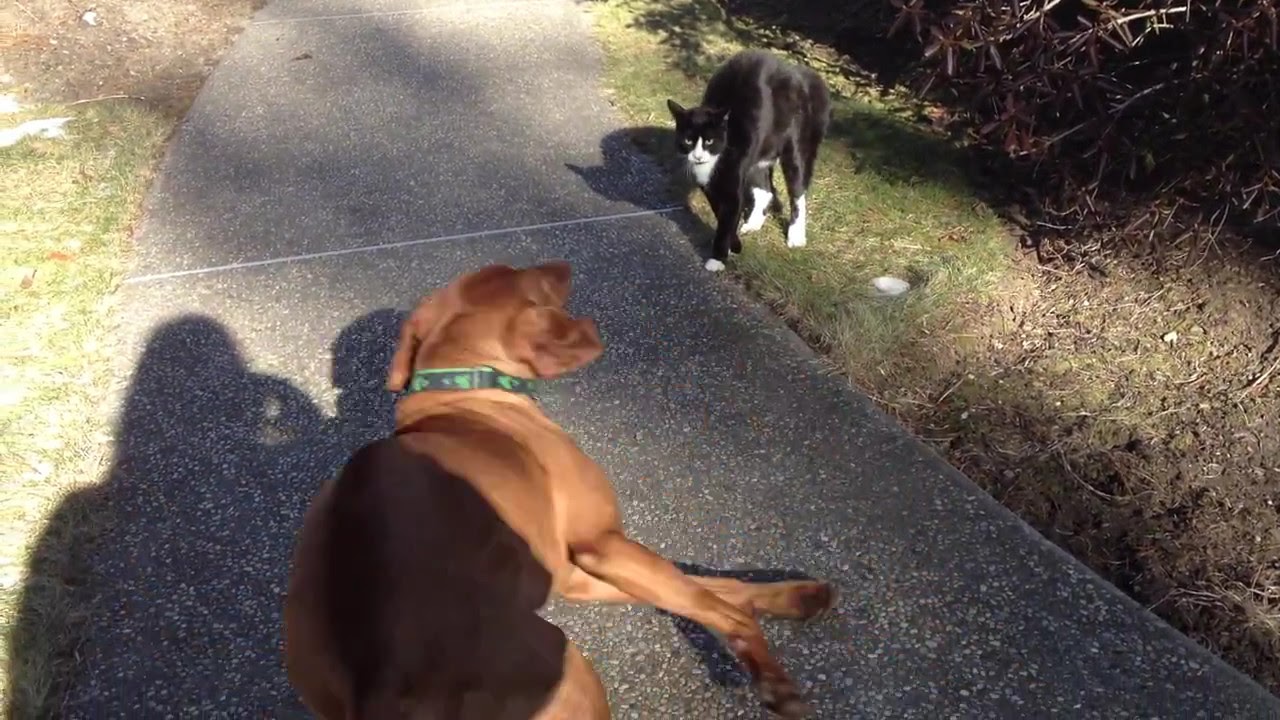The image depicts a dynamic scene on a sidewalk bordered by patches of grass and some scattered twigs. At the center, a small brown dog, possibly a dachshund with a green collar, is seated but appears alert and ready to move. Directly across from the dog, a black and white cat stands with its back slightly arched, suggesting a heightened state of attention or agitation. The cat gazes straight into the camera. The shadows of the individuals taking the photograph are visible on the left side of the frame, indicating that at least one of them is likely a female. The interplay of the animals' postures and the setting creates a captivating, almost tense moment captured in a suburban environment.